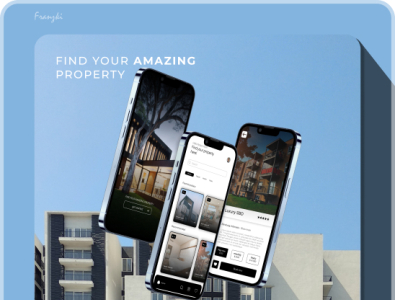This advertisement aims to help individuals find housing or a place to live. It features a design with two sky-blue squares. The larger outer square has partially legible white text in the upper left-hand corner, possibly beginning with an "F" and ending with "L I." The inner square, placed within the larger square, prominently displays the text "FIND YOUR AMAZING PROPERTY" in capital white letters in its upper left-hand corner.

Below this text are three smartphones, each showcasing different aspects of potential properties. The left phone displays an image of a house with a tree in front, with the inside room visibly lit up. The middle phone shows photos of a room and possibly other areas of a building. The right phone features an image of a multi-story apartment building with a visible star rating. The background behind these phones displays a building with a combination of white and navy blue walls, possibly an apartment complex.